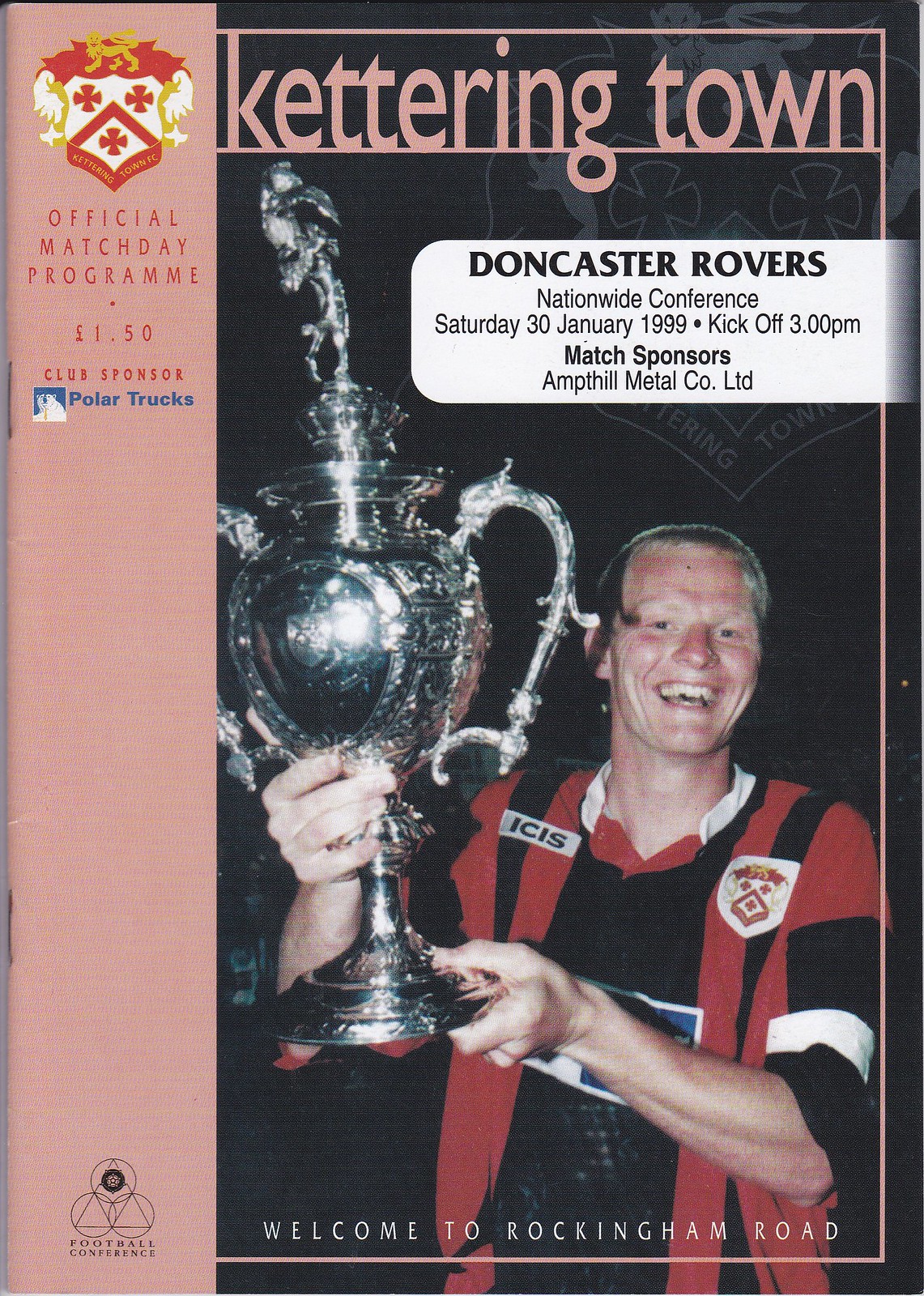This image depicts a vintage front cover of the official Match Day program for Kettering Town, priced at £1.50, now considered a collector's item. Dominating the cover is an ecstatic gentleman wearing a red and black striped football jersey, triumphantly hoisting an ornate, large silver trophy above his head with both hands, a broad grin plastered on his face. The top features peachy beige lettering spelling out "Ketteringtown," while a white bubble below displays "Doncaster Rovers." On the left side, there's a pink column showcasing a heraldic shield adorned with a lion and four-leaf clovers, possibly the team's logo. The bottom of the cover reads "Welcome to Rockingham Road."